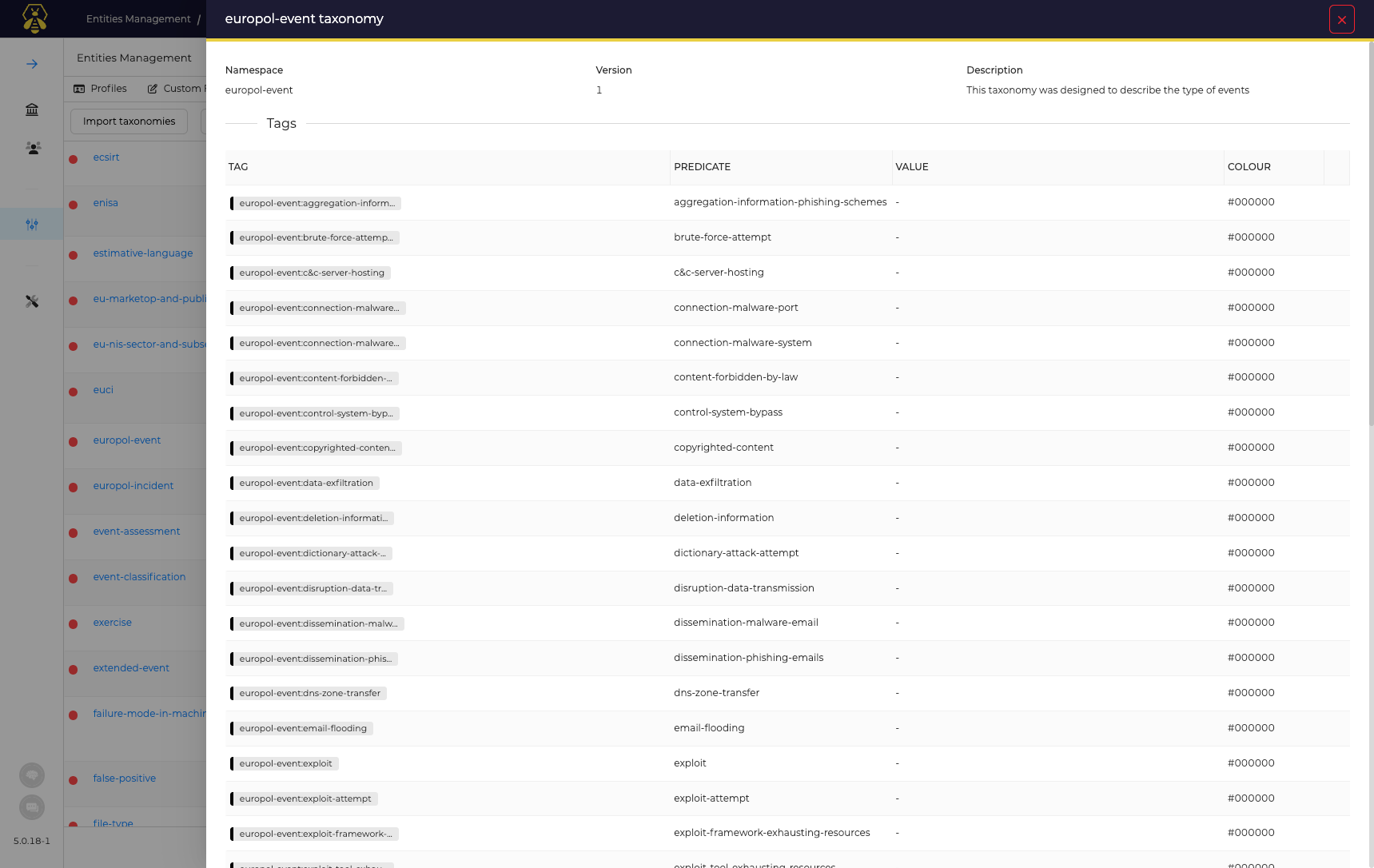This image, set against a stark white background, depicts a screenshot featuring numerous elements pertinent to Europol Event Taxonomy. At the very top, a black banner horizontally spans the image, adorned with contrasting white and yellow text. In the upper left corner, a distinctive yellow "B" logo is prominently displayed. To its right, small gray text reads "Entities Management / Europol Event Taxonomy."

Moving downward, a white rectangular box contains black text. It initially outlines, from left to right, "Namespace: Europol Event Version 1" and then continues with a "Description: This taxonomy was designed to describe the type of events." 

Directly below this, a light gray horizontal line appears, inscribed with the word "Tags." A subsequent row of tags runs vertically, one example being "Europol Event Aggregation in Form."

Additionally, there are two more columns presented across the screenshot. One is titled "Predicate Value," positioned in the middle, and to the far right is the final column labeled "Color."